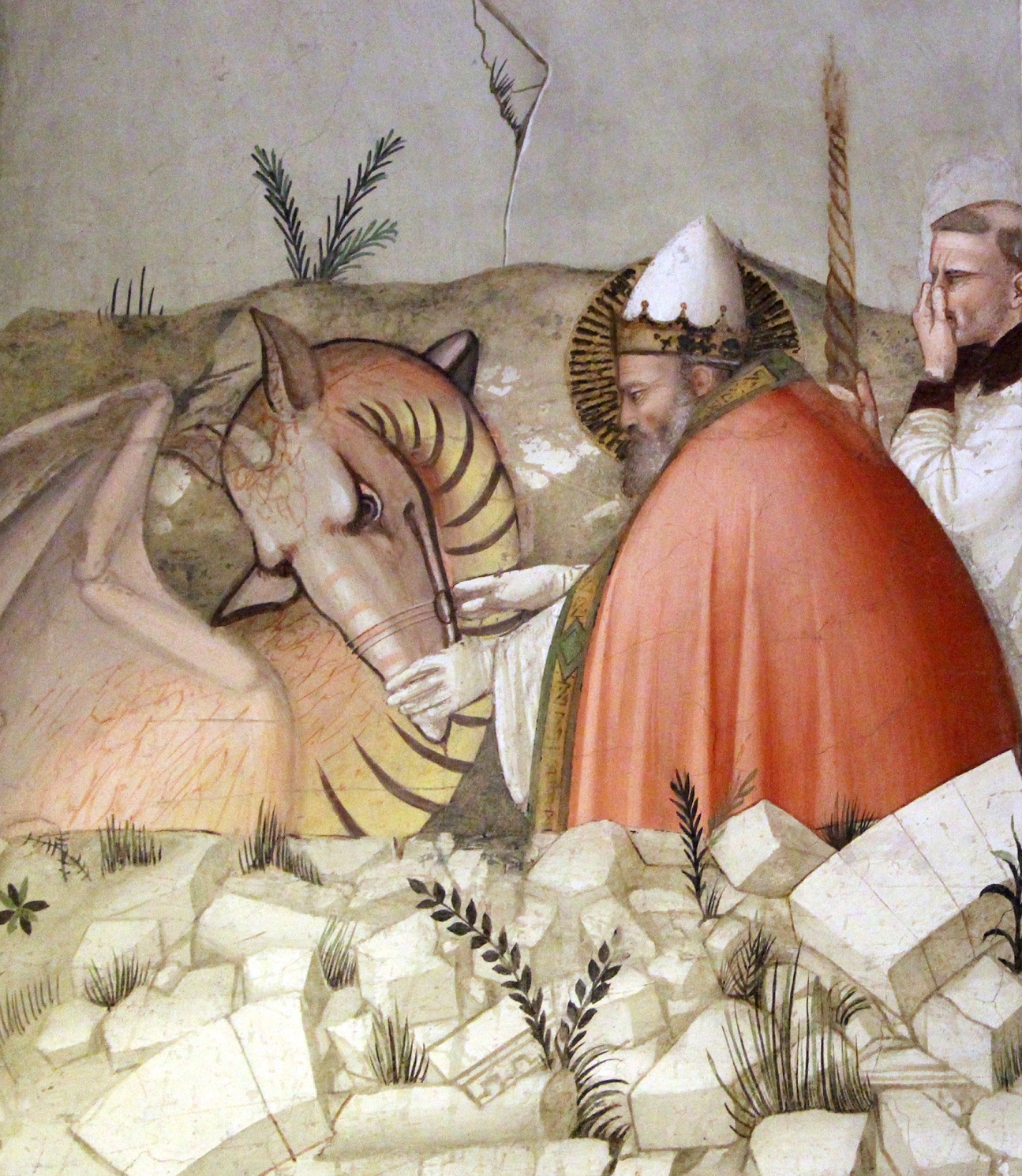The painting depicts a revered religious figure, possibly a bishop or pope who is recognized as a saint. The saint, notable for his long whitish-gray beard and golden halo, is clad in intricate liturgical garments, consisting of a red cloak with golden edges and white gloves. He wears a white mitre adorned with a golden crown. The painting captures a dramatic scene where the saint appears to be subduing a dragon. The dragon is an intriguing creature with light reddish-brown skin, black ridges on its belly, and peculiar horse-like ears; it looks menacing with its wings spread and horns projecting. To the saint’s right stands a monk or friar dressed in a black-and-white habit, identifiable by his tonsure. The friar is closing his eyes and pinching his nose, suggesting a foul smell in the scene. The foreground is strewn with broken white bricks interspersed with some green plants growing through the debris, adding to the dramatic and somewhat chaotic backdrop.